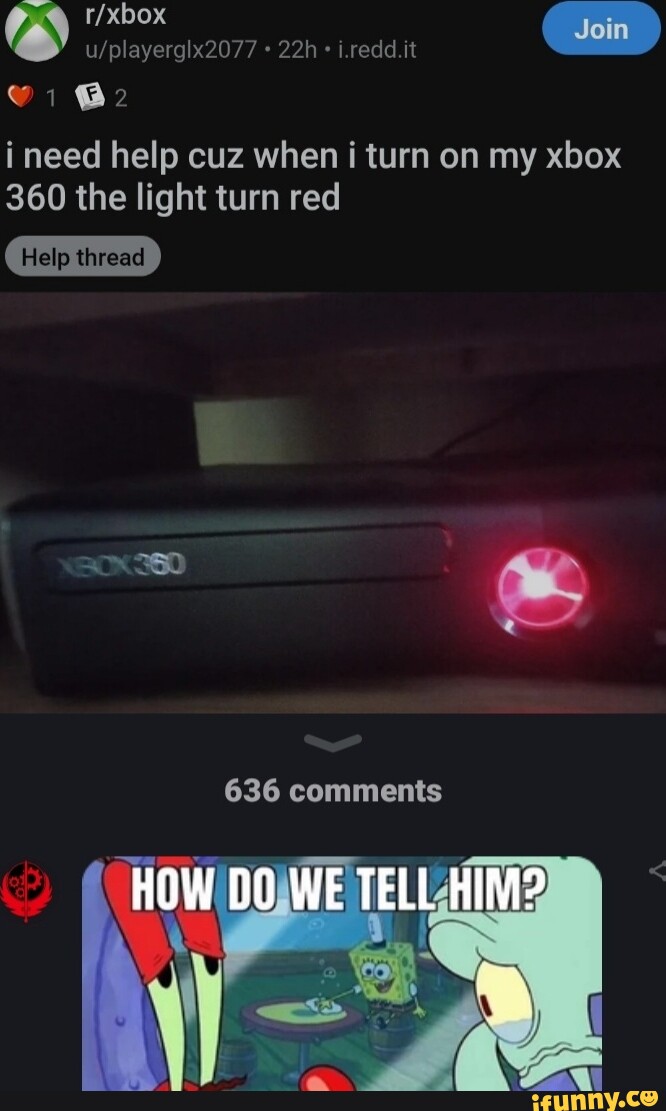A detailed screenshot from a Reddit mobile app displays a post from the r/Xbox subreddit by user u/player_glx2077, posted 22 hours ago. The interface includes a black background with a white circle featuring a green "X" in the upper left corner. Immediately to the right of this circle is the subreddit name "r/Xbox." Below the username, there is a blue "Join" button. Underneath this, a red heart icon with the number "1" beside it signifies one like, followed by a white comment icon with the letter "F" and the number "2," indicating two comments.

The central text reads: "I need help because when I turn on my Xbox 360, the light turns red." Below this plea, there's a gray "Help" button. The user has included an image captioning their post: a photograph of their black Xbox 360 console with an ominous red light shining, suggesting a system error.

A gray drop-down arrow follows this image, leading to a display that notes "336 comments" on the post. Additionally, someone has responded with a meme originating from SpongeBob SquarePants. The meme features a blurry background of SpongeBob and Mr. Krabs, with Mr. Krabs' eyes prominently on the left and what seems to be Squidward on the right side. The text overlay on the meme humorously asks, "How do we tell him?"